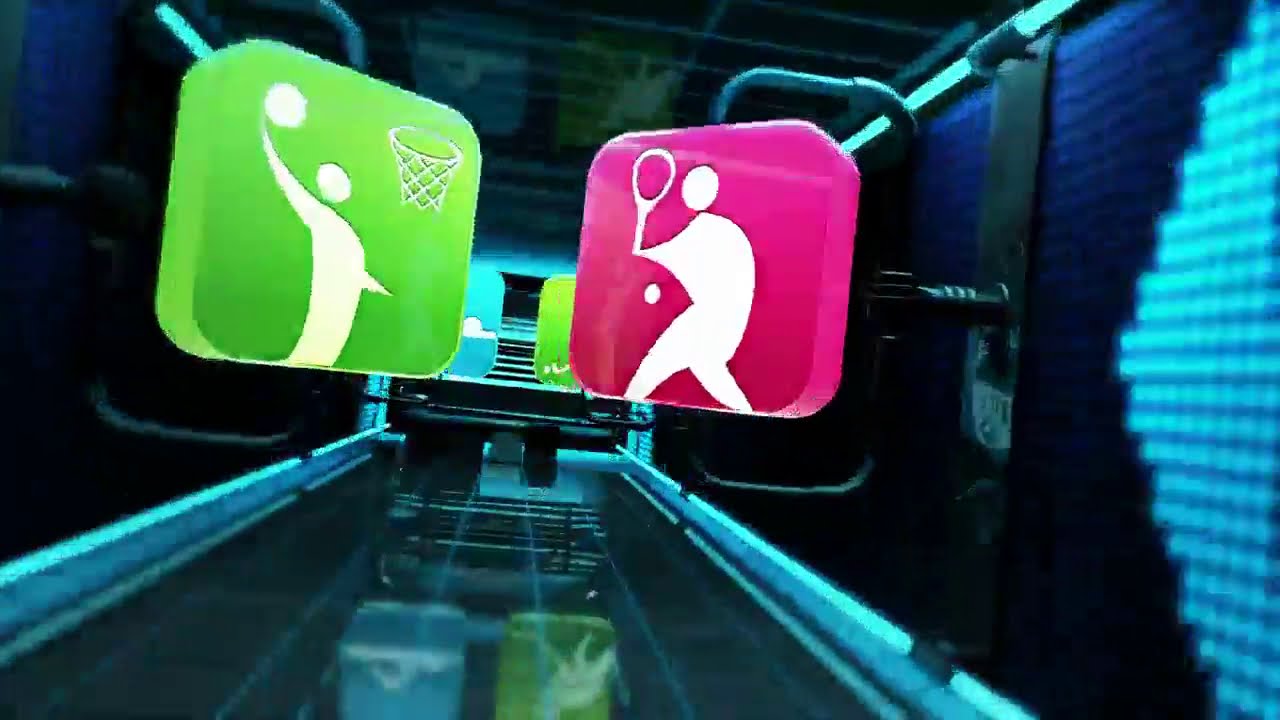The image appears to be a digitally animated scene set in a high-tech, futuristic hall or internal area of a device. The room features dark blue and black walls, a black ceiling, and a reflective, tiled floor lined with bright blue, glowing lines that resemble laser beams. Metal runners and bars, possibly for sliding or mounting objects, stretch across this space, enhancing the intricate technological aesthetic.

In the foreground, there are two prominent, colorful 3D logos or icons. The logo on the left is a green 3D box displaying a stylized, white cartoon figure about to dunk a basketball into a net situated to its right. The logo on the right is a bright pink 3D square, featuring a similar cartoon figure holding a tennis racket, seemingly about to hit a tennis ball. Both figures are simplified, abstract representations of human forms engaging in sports activities.

Behind these primary icons, the background contains additional, partially obscured buttons or logos of a similar style, hinting at further interactive elements or icons hidden in the scene. To the right side of the image, there are shapes that step upwards and back, composed of turquoise squares, adding depth and dimension to the setting. The overall composition is vibrant and dynamic, likely intended to advertise or promote a website, game, or sports-related content.